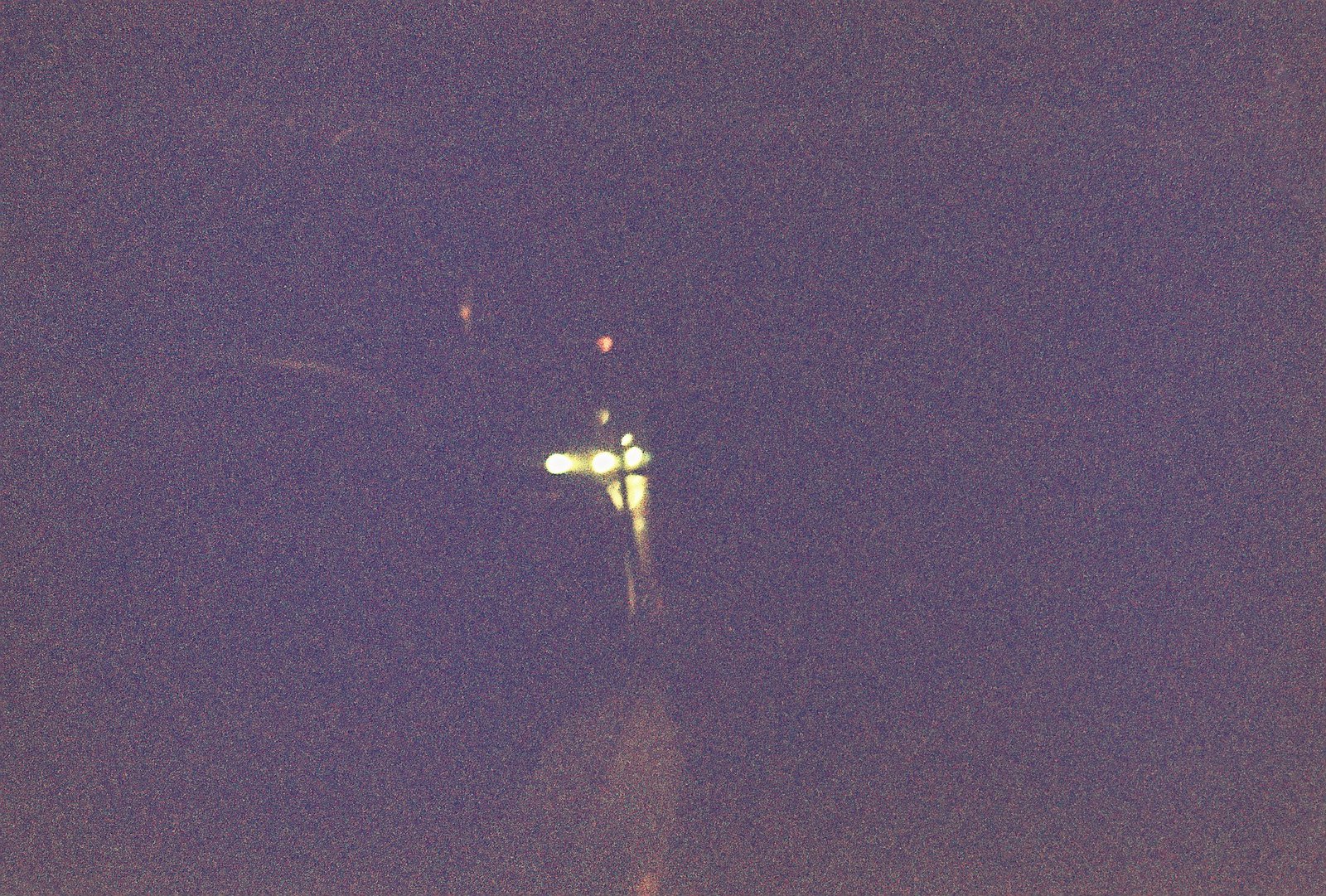The image is a grainy, dark nighttime shot with a predominant dark blue or purple tint, featuring pixelation throughout. Central to the image is a curved structure, potentially a bridge or pier, illuminated by several lights. Two prominent lights, possibly street lamps, are situated along its top. In the middle of the photo, an arrangement of light sources can be observed: a pair of car headlights, with a third light slightly behind them, and three larger white lights positioned in a row. Additionally, there are red circular lights, one to the left and one underneath, interspersed among the white lights. In the immediate foreground stands a cement barrier, and near the bottom center, a bright whitish rectangle with a pointed, sword-like shape. The brightest and most distinct lights are of varying sizes and positions, suggesting complex lighting either from vehicles or structured components against the otherwise blotchy and pixelated backdrop.